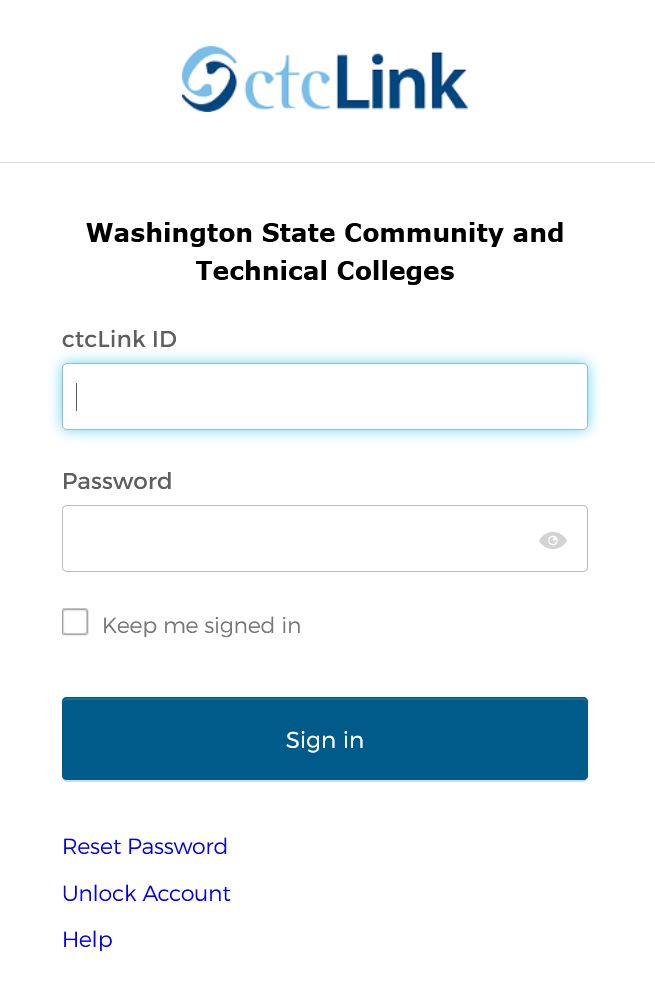Screenshot: Mobile Interface of CTC Link Login Page

The screenshot appears to capture a mobile interface of the CTC Link login page. The top of the screenshot features a white background displaying the text "Oh Something" alongside a link. Below, the interface showcases a light blue and dark blue circular pattern in the center. Within the light blue circle, it displays "CTC," and within the darker blue circle, it shows "Link" with a capitalized 'L'.

Further down, in bold black text, it reads "Washington State Community and Technical Colleges." On the left-hand side, in gray text, it says "CTC Link ID," with an adjacent entry field highlighted in blue for user input. Below this is another gray text field labeled "Password," which is empty, followed by an eye icon that allows users to toggle the visibility of their password. A checkmark appears next to the option "Keep me signed in."

At the bottom, a large blue rectangle features the "Sign In" text centered in white. Underneath this button, on the left-hand side, blue text links to "Reset Password," "Unlock Account," and "Help."

This detailed description encapsulates the entire CTC Link login interface as captured in the screenshot.